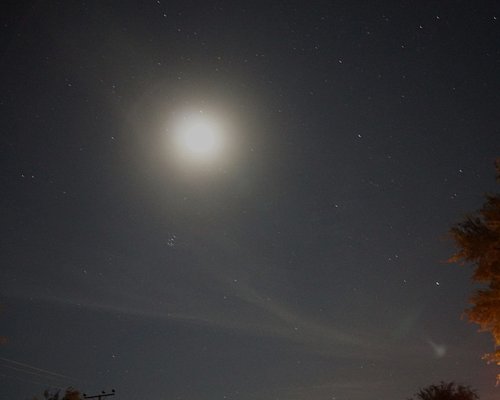The image captures a dark nighttime sky in a deep purple hue, sprinkled with slightly blurred white stars, indicative of their motion during the camera's exposure. A prominent round white sphere, presumably the moon, is situated towards the left-center of the image. The moon radiates a soft white corona that fades into the surrounding sky. Wispy clouds gently drift beneath it, barely discernible against the night backdrop. Thin, faded white lines, resembling jet trails, stretch across the sky. At the bottom of the image, the tops of two trees are visible, one with green leaves and the other with a canopy of orange leaves. Additionally, a telephone pole with extending wires is discernible, contributing to the scene’s sense of depth. On the right edge, there's a partial view of a tree with a brownish canopy. The overall composition provides a serene yet detailed snapshot of a nocturnal landscape.